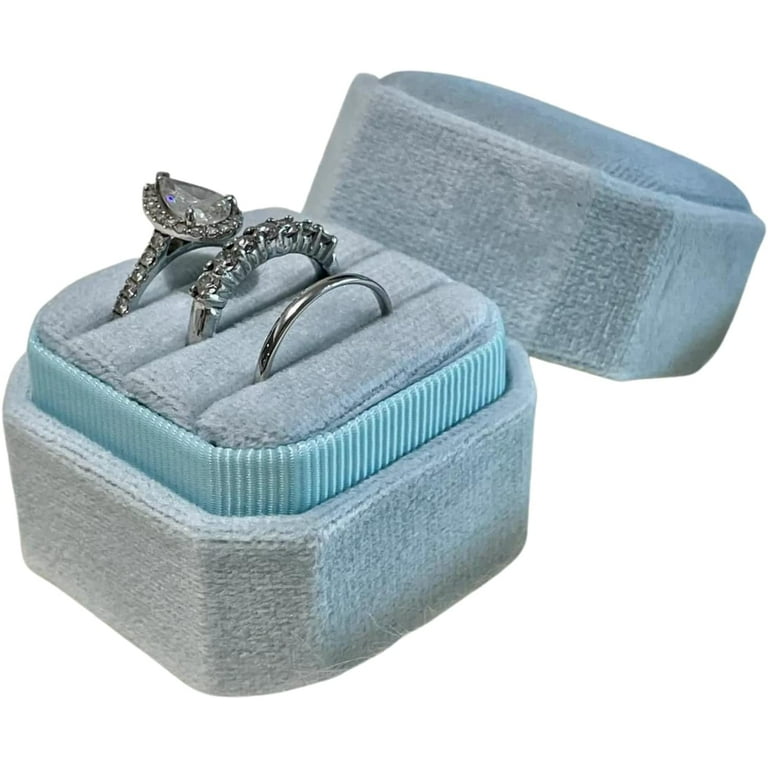The photograph depicts a luxurious powder blue velvet ring box with an open lid, revealing a felt-lined, piped baby blue pattern interior. Inside, the box features a hexagonal ring holder with three slots designed for rings. The first slot contains a simple silver or platinum band, modest and unadorned, resting halfway out of its holder. The ring in the second slot is slightly thicker, embellished with seven diamond or cubic zirconia insets arrayed along the top of the band. The third slot houses a dazzling engagement ring, nearly the same width as the first band but far more elaborate, adorned with a halo of diamonds along the band, culminating in a teardrop-shaped inset with a large, prominent diamond. The background of the image is white, emphasizing the elegance and details of the rings and the box.